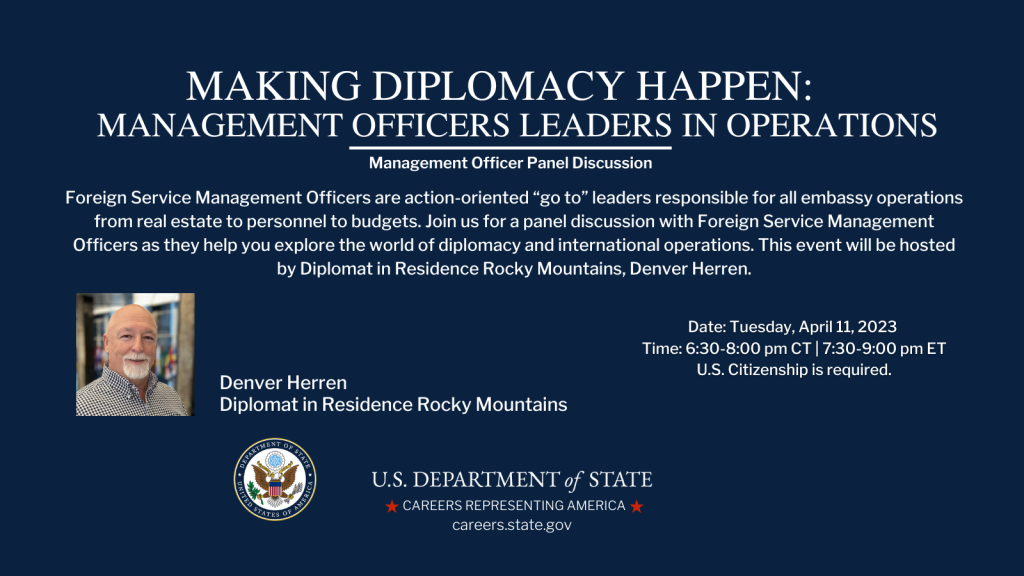The image is an advertisement with a dark navy blue background, featuring white text and the U.S. Department of State logo with an eagle at the bottom center. The headline reads "Making Diplomacy Happen" prominently at the top center. Below it, in slightly smaller font, it continues with "Management Officers, Leaders, and Operations" and "Management Officer Panel Discussion". A detailed paragraph explains that "Foreign Service Management Officers are action-oriented go-to leaders responsible for all embassy operations, from real estate to personnel to budgets."

To the left, there's a photograph of an older gentleman with a white beard identified as "Devin Herron, Diplomat in Residence, Rocky Mountains." The event details are listed towards the right of his image: "Date: Tuesday, April 11, 2023, Time: 6:30 to 8 p.m. CT, 7:30 to 9 p.m. ET." It also notes that "U.S. citizenship is required." The bottom of the image includes the text "U.S. Department of State, Careers Representing America," with the URL "careers.state.gov."